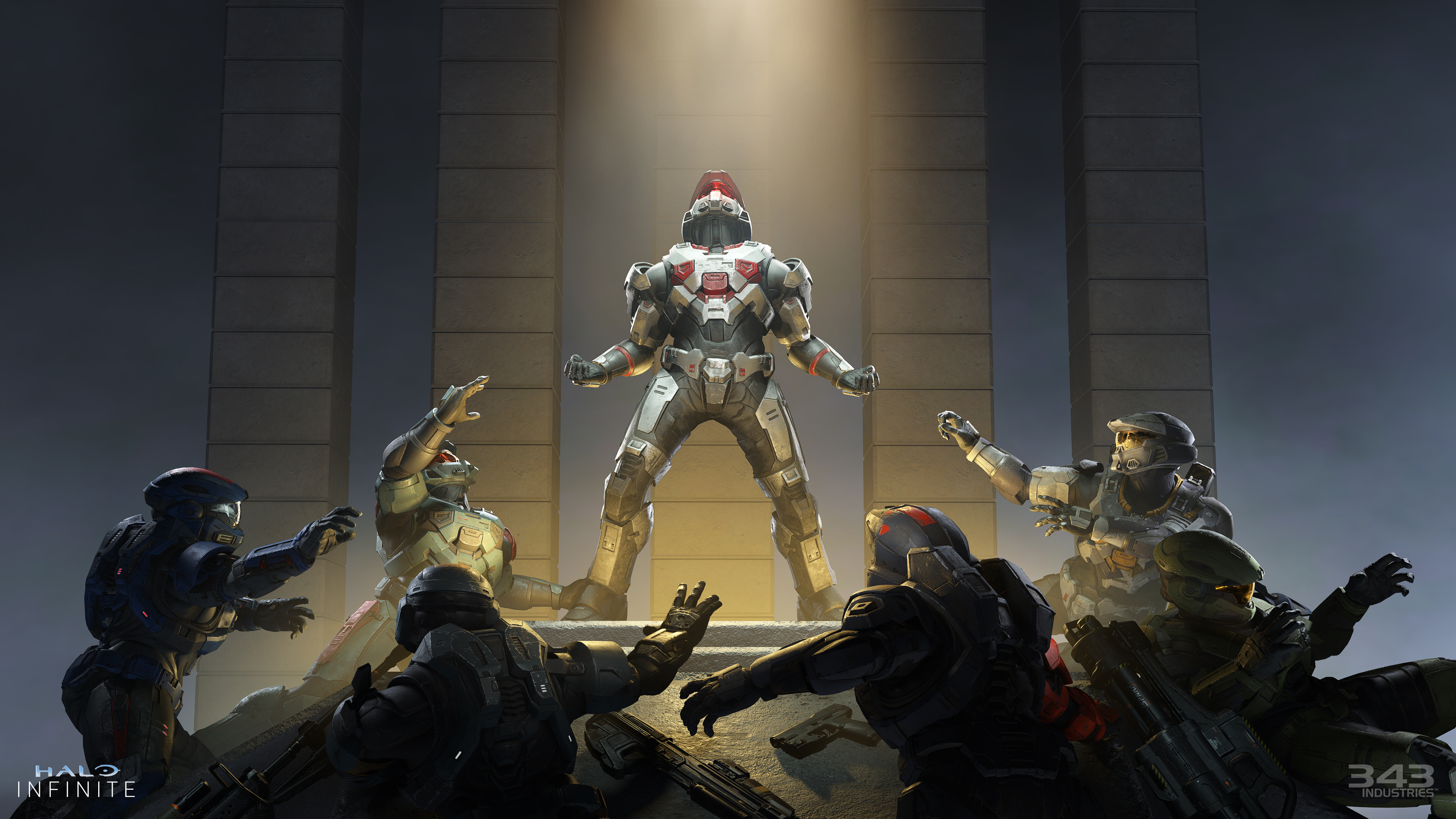The animated image, likely a screenshot or loading screen from the video game Halo Infinite, prominently displays the game's title in the bottom left corner and the developer, 343 Industries, in the bottom right corner. Central to the image is a Halo Spartan, clad in a high-tech suit reinforced with metal and plastic armor, standing with his hands clenched and looking upwards. Surrounding him are fellow Spartans in identical suits, complete with helmets accented in red. The background features a variety of weapons, including a noticeable handgun. The entire scene is brightly lit, showcasing the image's high clarity and detailed textures. The composition and lighting emphasize the group of Spartans amidst their advanced battlefield gear, highlighting the game's futuristic and immersive atmosphere.